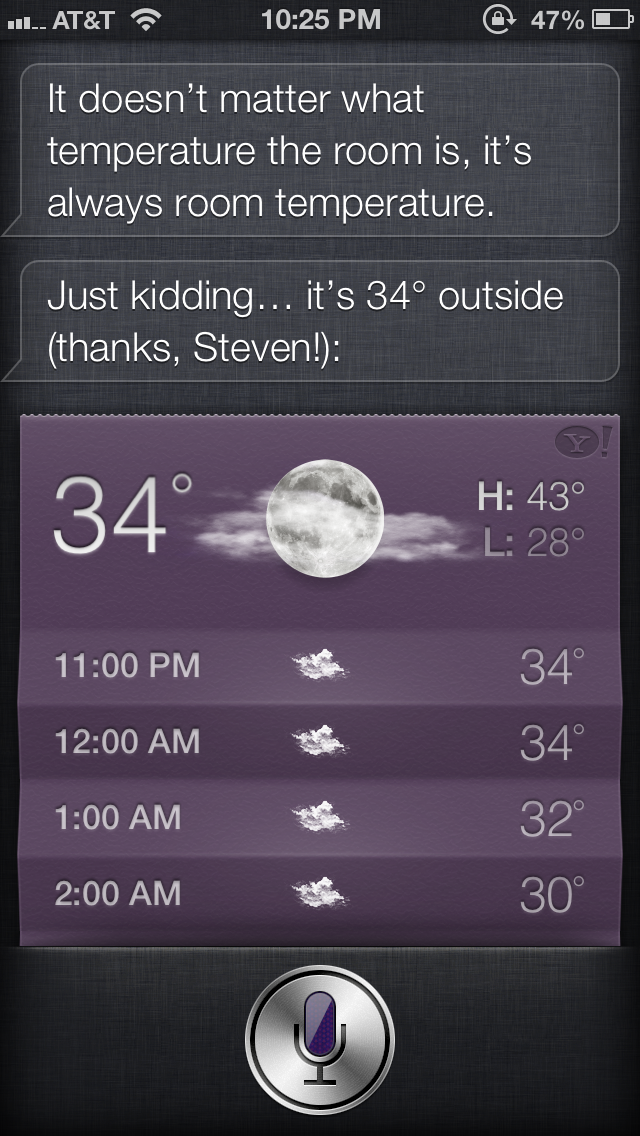The screenshot on the cell phone's screen captures a succinct yet detailed weather forecast and text conversation. At the top, the status bar reveals it's 10:25 p.m. with a 47% battery and AT&T signal strength. The text chain displays a lighthearted message from Siri stating, "It doesn't matter what temperature the room is. It's always room temperature," followed by, "Just kidding, it's 34 degrees outside. Thanks Steven." Below, a weather widget shows a moon icon indicating clear skies with a temperature of 34 degrees, a high of 43 degrees, and a low of 28 degrees. The forecast predicts 34 degrees at 11 p.m. and 12 a.m., 32 degrees at 1 a.m., and 30 degrees at 2 a.m., all displayed along with a little microphone button at the bottom center for text-to-speech input.